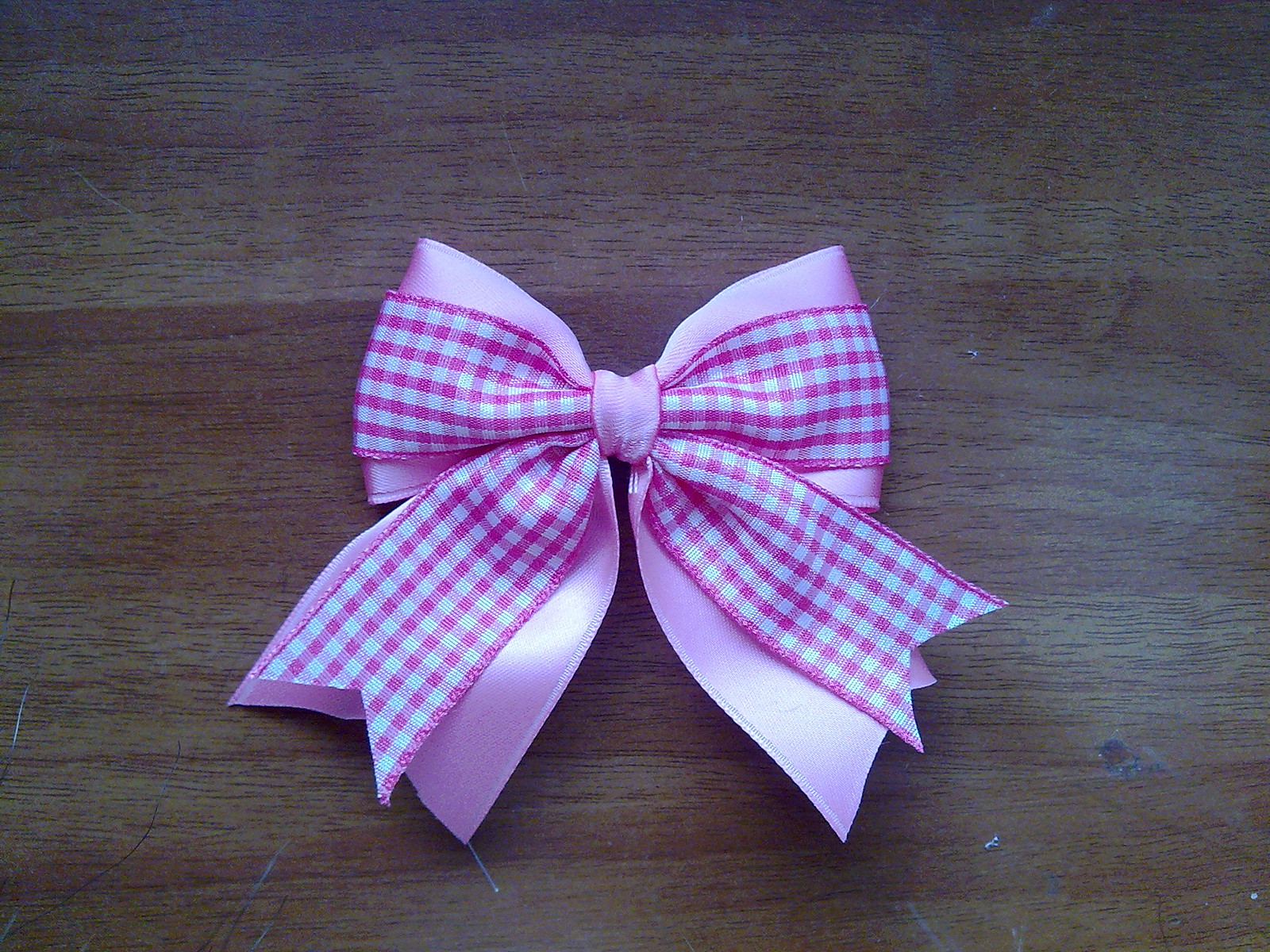The image features a dull, medium brown wooden floor with visible variations in the grain and texture, giving it an aged and scuffed appearance with multiple scratches and possible stains. In the center of this floor rests a delicate ribbon bow. The bow is primarily light pink with a checkered design in pink and white on the top layer and solid light pink underneath. The checkered pattern is composed of thin, vertically and horizontally striped lines, creating a subtle checkerboard effect. The bow has a symmetrical, tidy appearance, almost resembling a bow tie, with two short tails extending to either side. The intricate layering of the ribbon and precise placement makes it a focal point of the image.